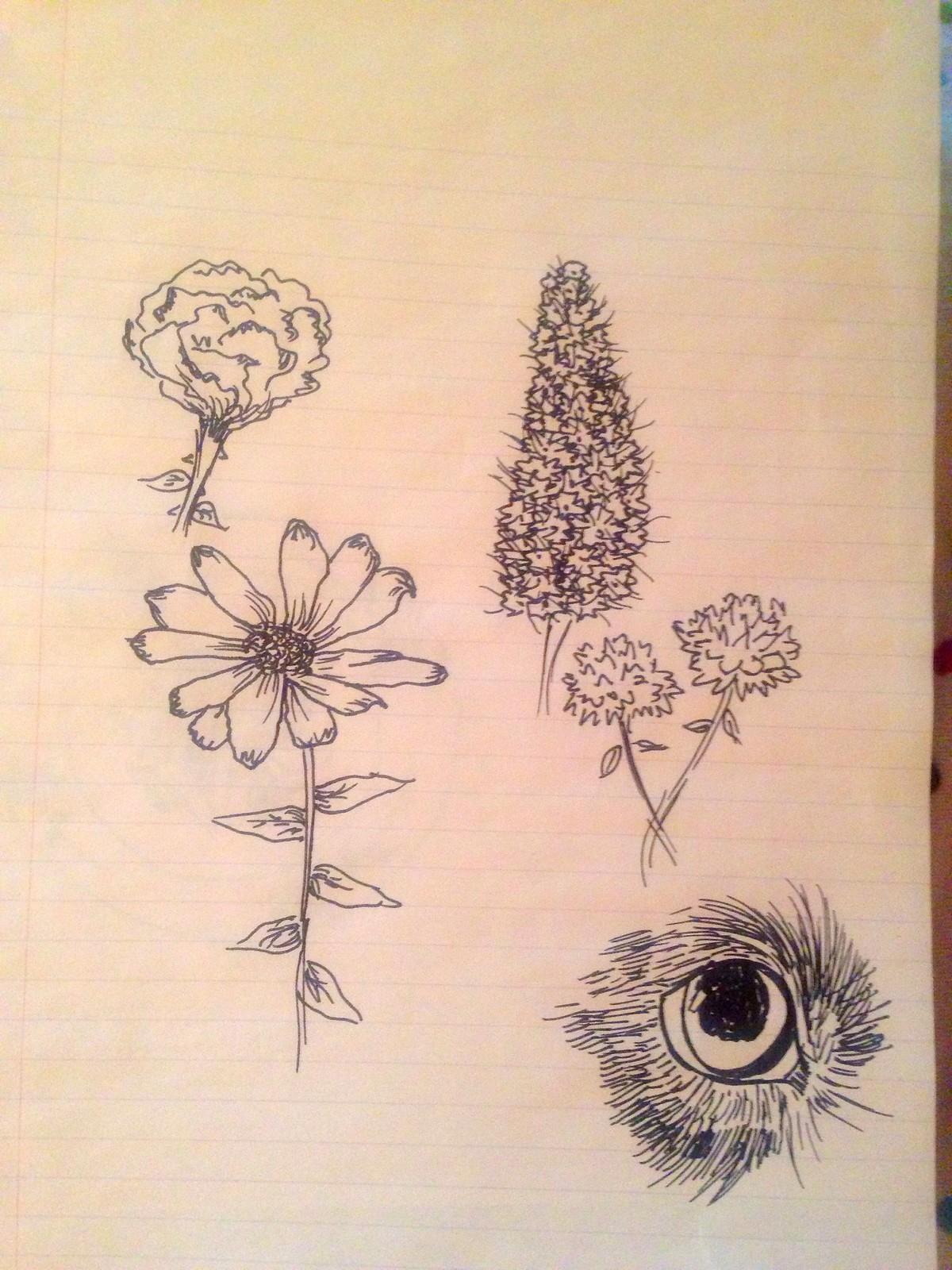The image is a detailed sketch on a piece of off-white, lined notebook paper with a faint red margin line on the left edge. The central and bottom sections of the page are filled with various drawings, seemingly created with black ink or possibly pencil. Starting from the top left, there is an illustration of an unopened flower with petals and leaves tightly bunched together, accompanied by a stem with small leaves protruding from each side. Directly below it is a larger, fully bloomed flower with a prominent pistil at the center, a thinner stem, and five larger leaves (two on the left and three on the right).

To the top right of the page is a sketch resembling a narrow tree with dense foliage that obscures the trunk and branches, giving it a corn-like appearance with roots peeking out below. Underneath this, there are two intertwined fuzzy flowers or plants, with stems crossing each other. Lower on the page, there is an intricately detailed eye of an animal, possibly a bird or an animal with black fur or feathers encircling the eye, with the dark pupil prominently visible. The placement of these elements appears random but centrally focused, suggesting a spontaneous, artistic doodle.